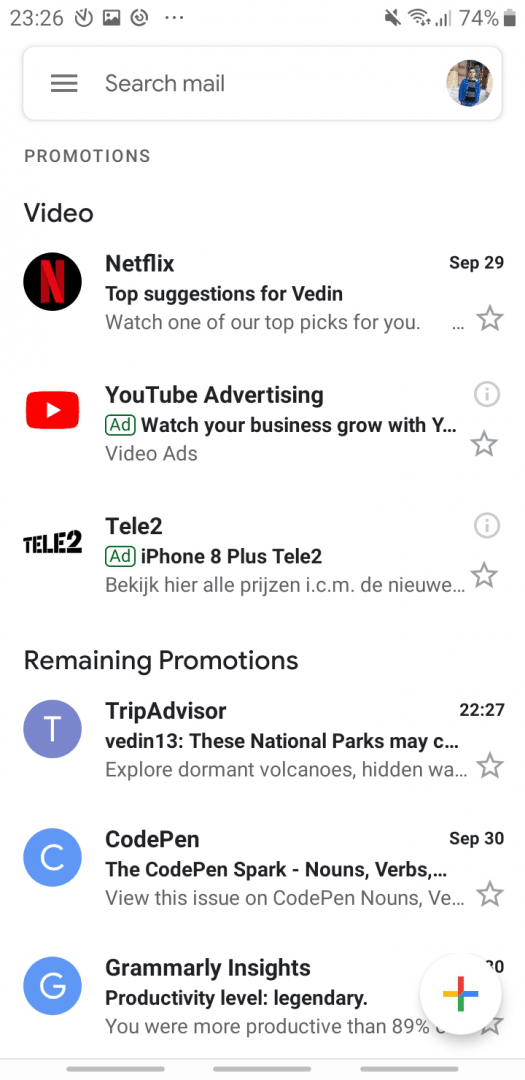A detailed cell phone screenshot captured at 23:26, as displayed on the upper left-hand corner. Beside the time, there are three icons including a screenshot icon and two circular icons with three horizontal dots. On the upper right-hand corner, the phone's ringer is turned off, with the Wi-Fi and cellular reception icons visible, and the battery level at 74%. Just below these icons is a search mail bar featuring a profile picture of a man wearing a blue coat. The screen shows the "Promotions" tab in an email application. Listed under "Promotions" are emails from "Netflix," "YouTube Advertising," and "Tele2." Further down, under "Remaining Promotions," emails from "TripAdvisor," "CodePen," and "Grammarly Insights" are visible.